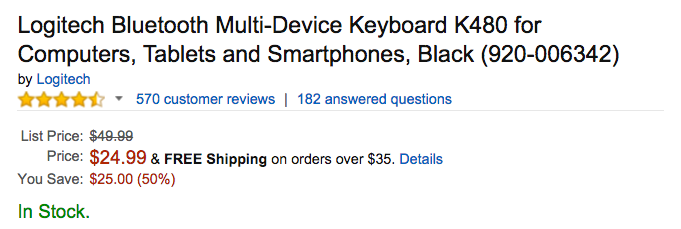**Logitech Bluetooth Multi-Device Keyboard K480 - Black | Model 920-0036342**

- **Compatibility:** Suitable for computers, tablets, and smartphones
- **Rating:** 4.5 stars based on 570 customer reviews
- **Customer Engagement:** 182 answered questions
- **Pricing:** Originally listed at $49.99, currently available for $24.99 (50% off, you save $25)
- **Shipping:** Free shipping on orders over $35
- **Availability:** In Stock (as indicated in green)
- **Description:** The Logitech Bluetooth Multi-Device Keyboard K480 is a versatile keyboard designed to work seamlessly with multiple devices. Its sleek black design makes it a stylish addition to any workspace. Please note, there are no images included with this listing. Take advantage of this great deal on a highly rated keyboard, perfect for enhancing your productivity across your devices.